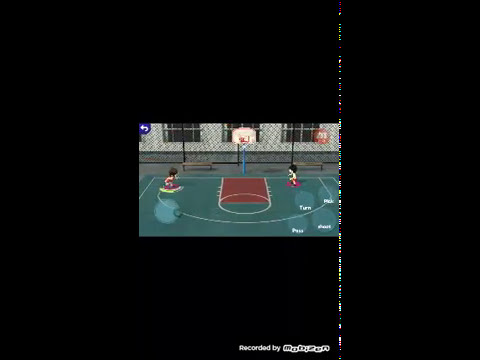This image appears to be a screenshot from an old video game or animation featuring a basketball court set against a pitch-black background, reminiscent of an old TV with picture interference. The court itself is a mix of turquoise and brown with white lines, accompanied by a single hoop mounted on a blue pillar with a white backboard and red rim, located in the upper right corner. Two brightly colored characters with black hair are positioned on the court, one on the left and one on the right. The ground features a green and red rubber mat, and each side has a bench bordered by a chain-link fence. In the background is a white building with three black windows. Scattered across the court are various turquoise objects, including what seem to be four round ones in the lower right corner and another in the lower left. Faded text overlays the image with options like "turn," "pick," and "pass." At the bottom, the caption "recorded by Mobizen" suggests the screenshot was captured using said software.